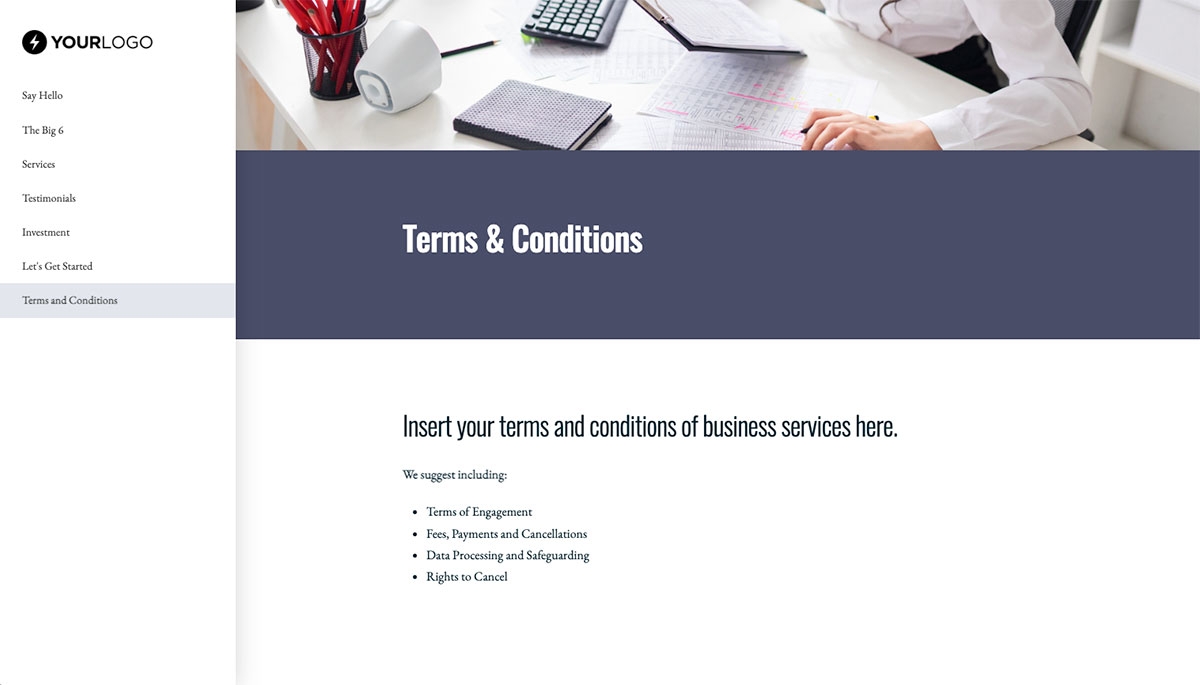The image depicts a webpage showcasing a work environment with various elements. At the forefront is a desk occupied by a woman wearing a white, long-sleeve shirt. She is engrossed in her work, holding a pen in her left hand and reviewing some papers. Her attention is directed towards a computer screen, visible alongside a keyboard. A pencil holder appears to have tipped over, scattering pencils, and next to it lies a potentially fallen coffee mug, also white. The desk is additionally cluttered with a book and more papers.

In the background, a white shelf complements the scene. The webpage displays sections with headers and text. Prominently, a section details "Terms and Conditions" in white text on a black background, advising that one should include terms of engagement, fees, payments, cancellations, data processing and safeguarding, and rights to cancel. To the left, a side bar hosts a navy blue circle featuring a white lightning bolt icon and is labeled with navigation options such as "Say Hello," "The Big Six," "Services," "Testimonials," "Investment," and "Let's Get Started," followed by a gray box with "Terms and Conditions." The webpage suggests it extends further than the visible area, indicating more content below.